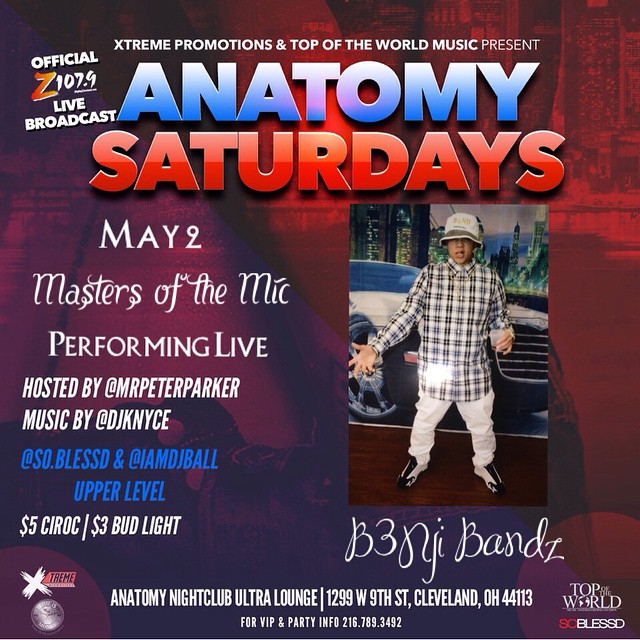This vibrant flyer for Anatomy Nightclub Ultra Lounge in Cleveland, Ohio, promotes an event titled "Anatomy Saturdays" with blue and red text. Presented by Extreme Promotions and Top of the World Music, the official Z107.9 live broadcast will feature the "Masters of the Mic" performing live on May 2nd. The event is hosted by Mr. Peter Parker with music by DJ KNYCE. Social media handles include @So.Blessed and @IAmDJBall, indicating their involvement on the upper level. The flyer also boasts $5 Ciroc and $3 Bud Light promotions.

On the right-hand side, there's a dynamic image of a man wearing a plaid black-and-white shirt, a bucket hat, white pants, and black-and-white sneakers, standing in front of a large Mercedes-Benz. His name appears in white cursive text, though it's hard to decipher. The address for Anatomy Nightclub Ultra Lounge is provided at the bottom: 1299 West 9th Street, Cleveland, Ohio, 44113. The background is predominantly a striking mix of red and purple.